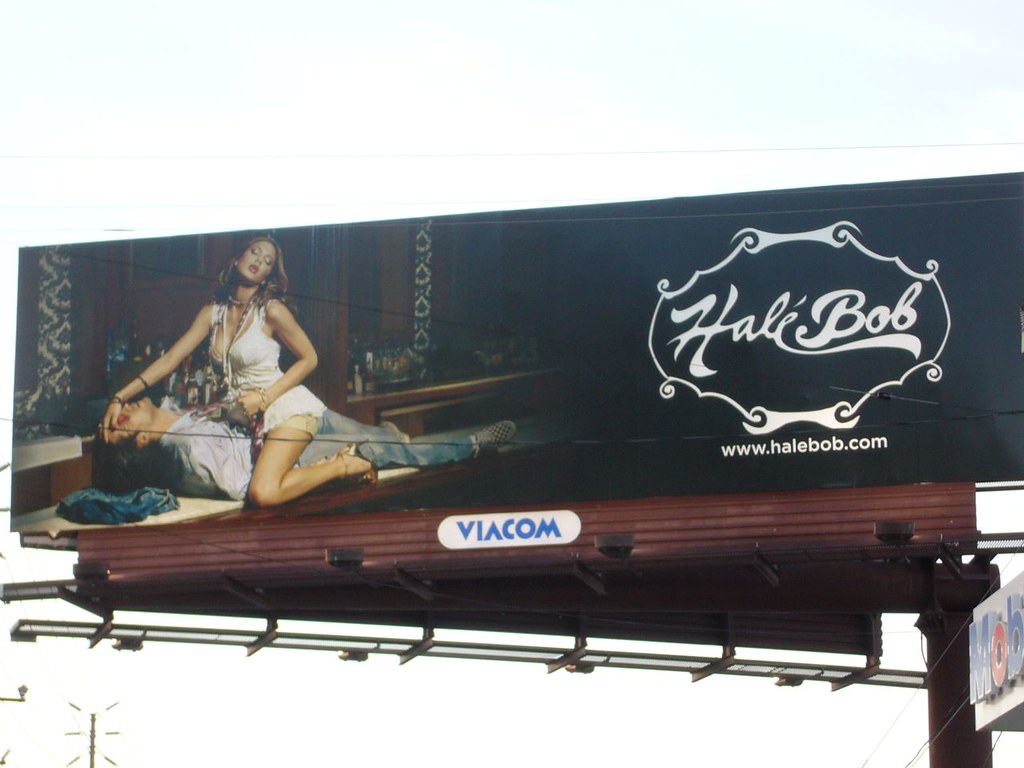The image showcases a provocative, rectangular billboard owned by Viacom, as indicated by their name at the bottom of the billboard's base. The main scene features a seductive, fair-skined woman in a very short white dress, adorned with necklaces, high heels, and offering a dreamy, seductive expression with her eyes closed. She is straddling a man, leaning back slightly with her right hand on his forehead and her left hand by her side, while holding him in place with her knees on his arms. The man, with his eyes also closed, appears to be lying under her spell, dressed in blue jeans, sneakers, and a white button-up shirt. The backdrop of the billboard is black, further emphasizing the white text "Hail Bob" along with its website, www.hailbob.com, emblazoned at the center-right, surrounded by a wave-like logo. The sky behind the billboard appears bright and white, and an additional partially visible sign with blue and red letters "M-O-B" is situated at the bottom right.